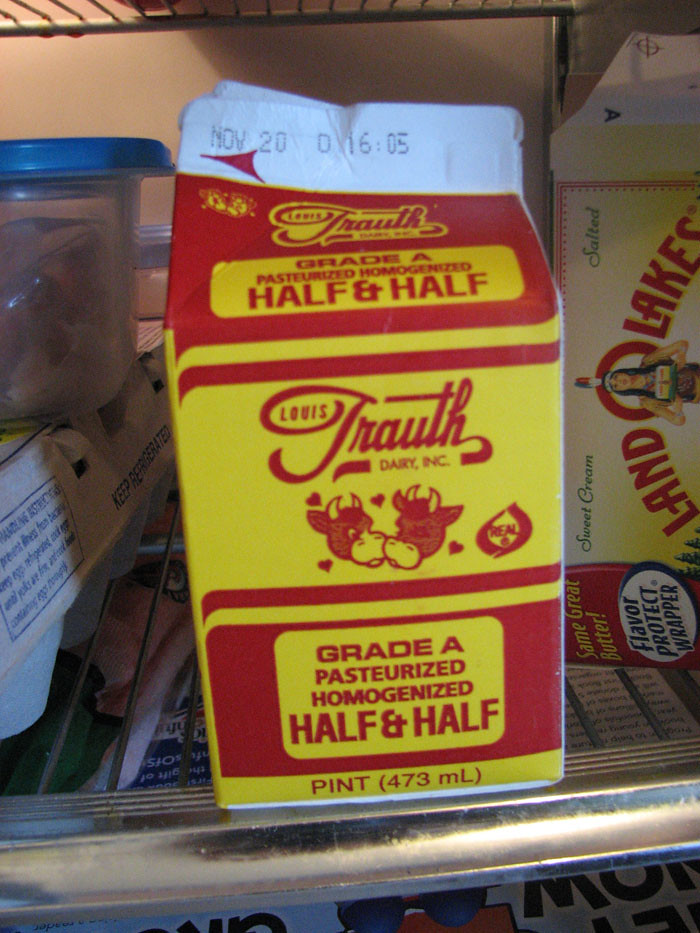A close-up photograph captures a meticulously arranged refrigerator shelf with a silver wire grate and edge. The focal point is a small pint carton of half-and-half with a vibrant red and yellow label. On the top ridge, an expiration date of November 20th is prominently displayed, along with a manufacturing time of 16:05. The carton is branded as Lewis Trouth Dairy, Inc., featuring Grade A, pasteurized, and homogenized half-and-half. The label showcases a traditional dairy emblem, a red "Real Dairy" symbol situated to the right of a middle logo depicting two horned Jersey cows with white muzzles touching noses. The right cow’s eyes are closed, while the left cow’s eyes are open, surrounded by four small hearts. At the bottom of the label, "Pint" is written in red text against a yellow background, with "(473 milliliter)" in parentheses. To the right of the half-and-half, a box of Land O' Lakes butter lies tilted on its side with the top partially open. On the left side of the shelf, a Tupperware container sits atop a large 12-dozen egg carton, adding a touch of everyday practicality to the composition.